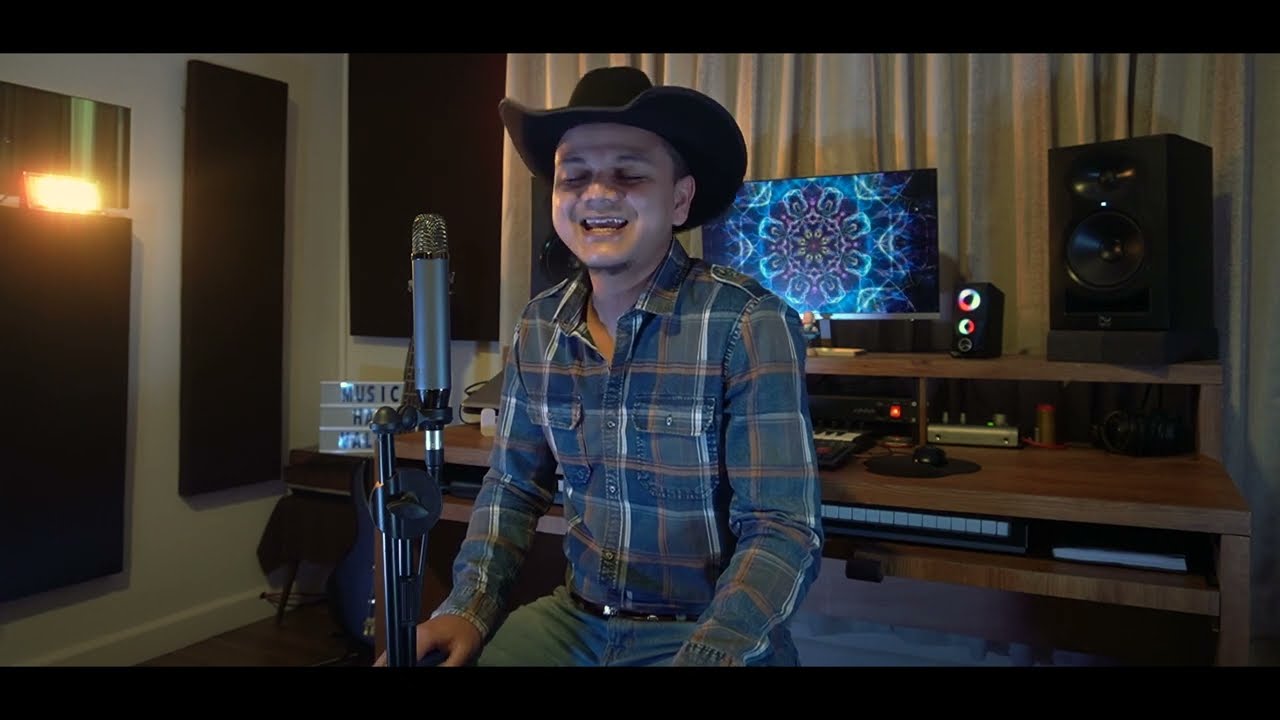In the image, a young man sits inside what appears to be a home office or music studio. He is facing the camera with a wide smile or laugh, eyes closed, wearing a black cowboy hat, a blue, brown, and white plaid shirt, and jeans. In front of him stands a silver microphone on a stand. Behind him is a light-colored wooden desk housing a computer monitor displaying a vibrant mandala design in purples and blues. To the right of the monitor sits a black speaker. The background features white walls adorned with long vertical black panels, possibly acoustic treatments, and thick white curtains. To the left of the man, there appears to be a guitar propped against the desk. The setting creates an atmosphere of a creative workspace or music studio.